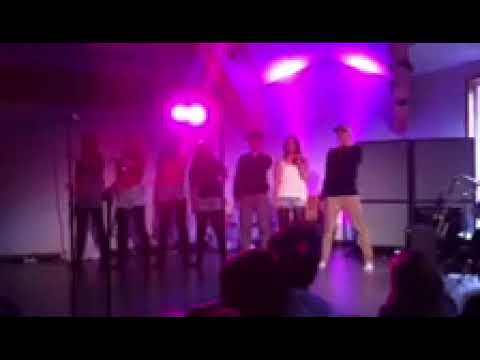In this highly pixelated and grainy photograph, we observe a group of people, possibly women with long hair, standing on a stage bathed in purple-hued lighting. The stage, which occupies the center and slightly off-left of the horizontal rectangular image, is flanked by a microphone stand on the left side. The lighting setup, situated above and behind the performers, contributes to the image's blurry quality, casting a colorful haze in shades of pink, blue, purple, orange, red, beige, white, black, and gray. The audience is located at the bottom right, evident by the visible heads. Although the exact number of performers is unclear due to the image's low quality, anywhere from four to eight individuals can be discerned, some of whom might be shadows. Additionally, a room divider with distinct panels is noticeable on the right side of the background, enhancing the impression of an indoor stage setting. This image likely captures a still shot from a video of a performance.